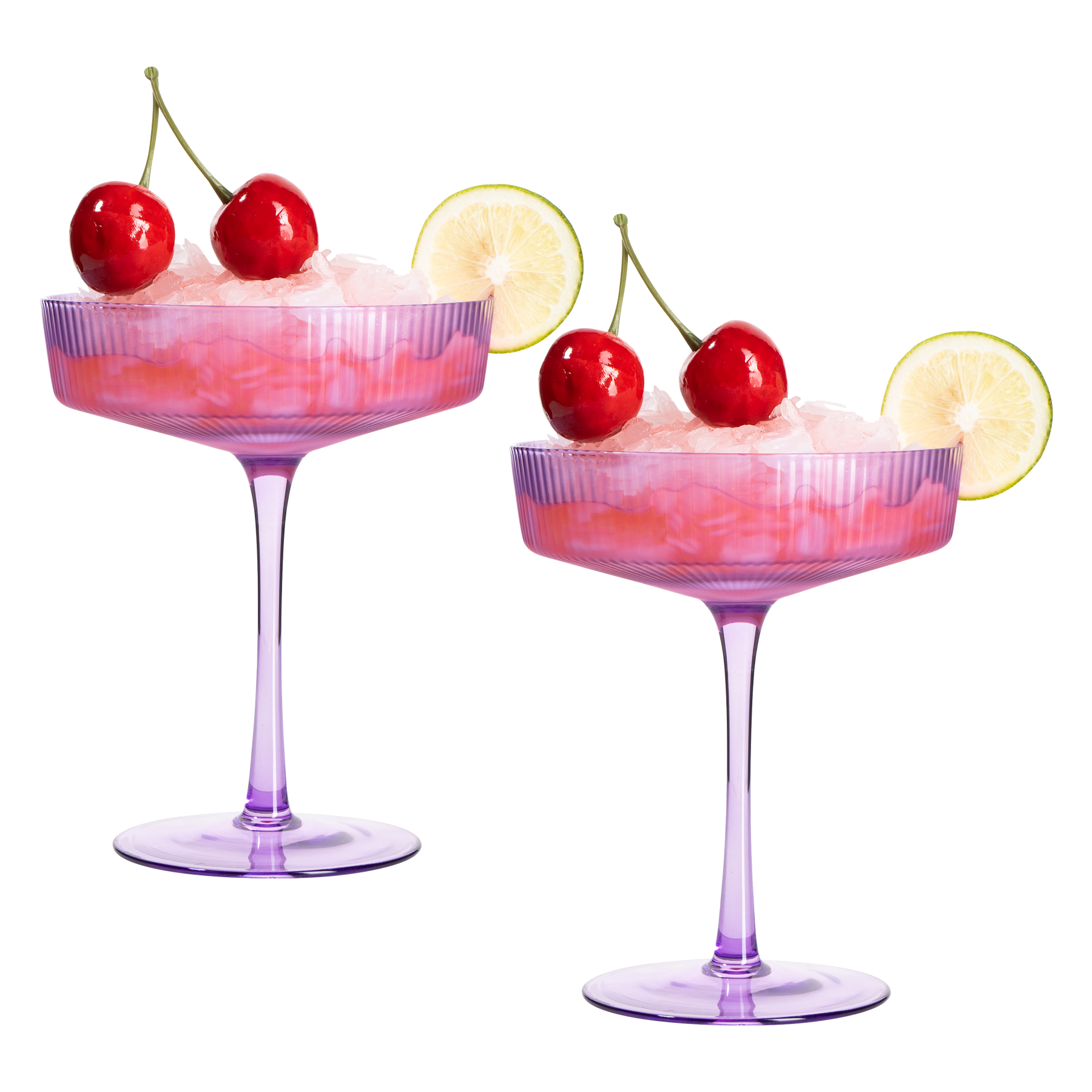The image depicts two identical mixed drinks presented in elegant, modern-styled, stemmed glasses that resemble traditional champagne glasses. Each plastic glass, colored purple, ends in an open-faced spherical base. The glasses are adorned with vertical lines for a touch of design. The drinks themselves consist of a layered, slushy concoction, displaying a gradient from white at the top to a light pink at the bottom. Floating ice is visible within the mixture. Atop each drink rests a set of twin cherries attached to a single stem, and a thinly sliced lime is placed on the rim of each glass. Although the glasses appear to be identical mirror images, the one on the left is slightly elevated compared to the one on the right. The backdrop of the image is completely white, emphasizing the colorful and meticulous details of the beverages.